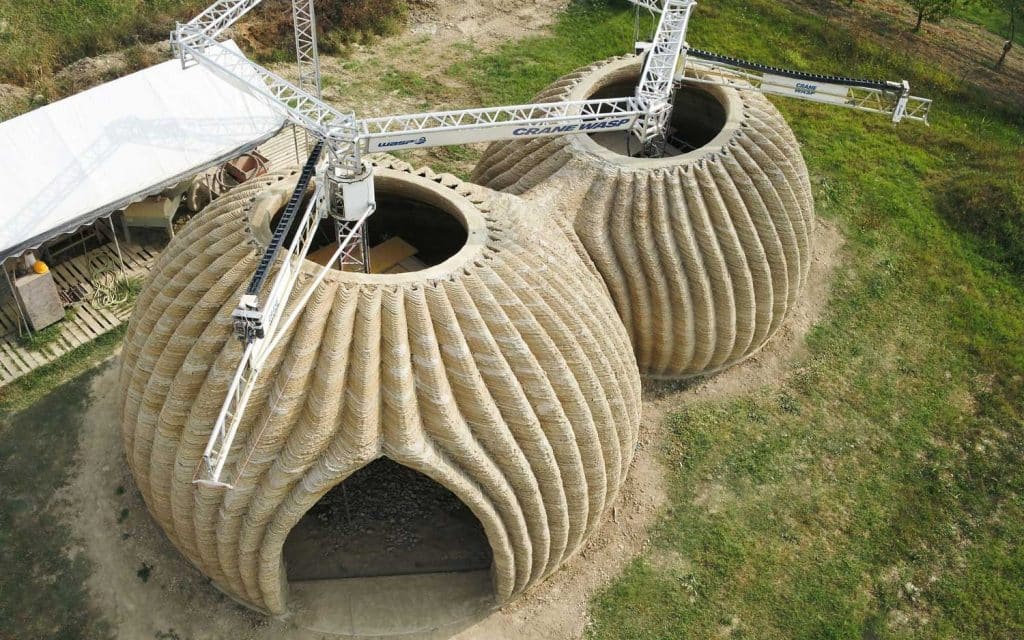The aerial landscape photograph showcases two large, round, beehive-shaped domes made of a material that resembles woven baskets or earth-toned natural fibers. These unique structures exhibit an accordion-like texture with ridges extending from the base to the roof. At the top of each dome are uniform, circular openings resembling Y-shaped propellers or crane structures, which protrude prominently. The domes are located amidst a field of green grass, and to the left, a white awning can be seen, possibly covering additional equipment or a pallet floor. The intricate details and unconventional architecture of the domes, labeled "crane wasp," add a layer of mystery, as their exact purpose remains unclear.